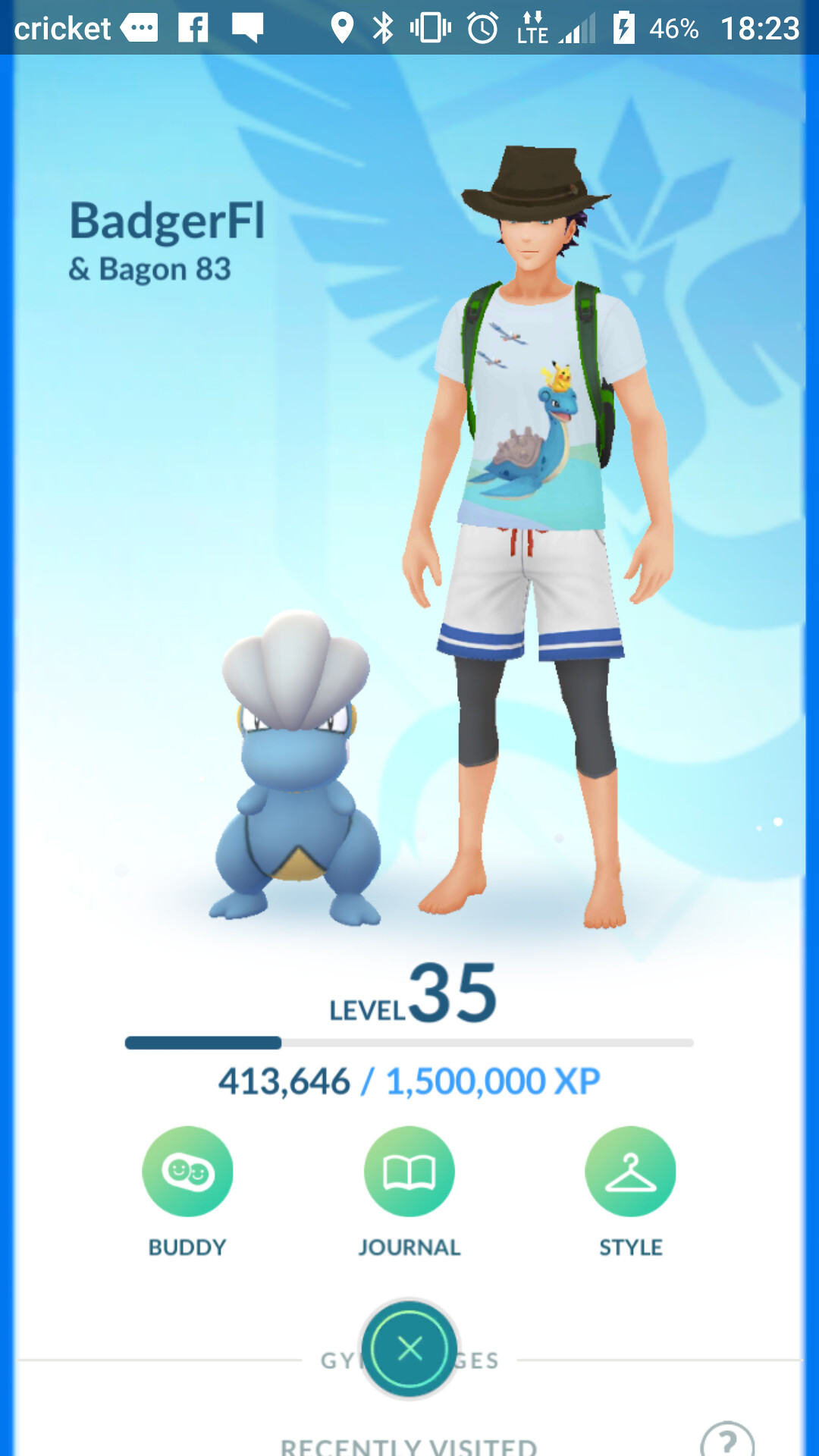The screenshot appears to be from a cell phone displaying the popular mobile game, Pokémon Go. The top of the screen features standard phone icons such as LTE connectivity, Wi-Fi, battery level at 46%, the time displayed as 18:23, and app notifications including the Facebook logo and Cricut service provider. The background transitions from light blue at the top to white towards the bottom. 

In the center-right of the screen stands a young male avatar. He sports a black fedora, a white T-shirt emblazoned with Pikachu and an aquatic Pokémon, white shorts, black knee pads, and is barefoot. Beside him to the left is a small blue Pokémon with a white shell-like head. 

Visible on the left side are the words "Badger Phi" and "Bagon 83." Below this text is a level bar indicating that the player is at Level 35 with 413,646 XP out of the 1,500,000 XP needed to advance to Level 36. At the bottom of the screen are three green circular icons labeled: Buddy, Journal, and Style.